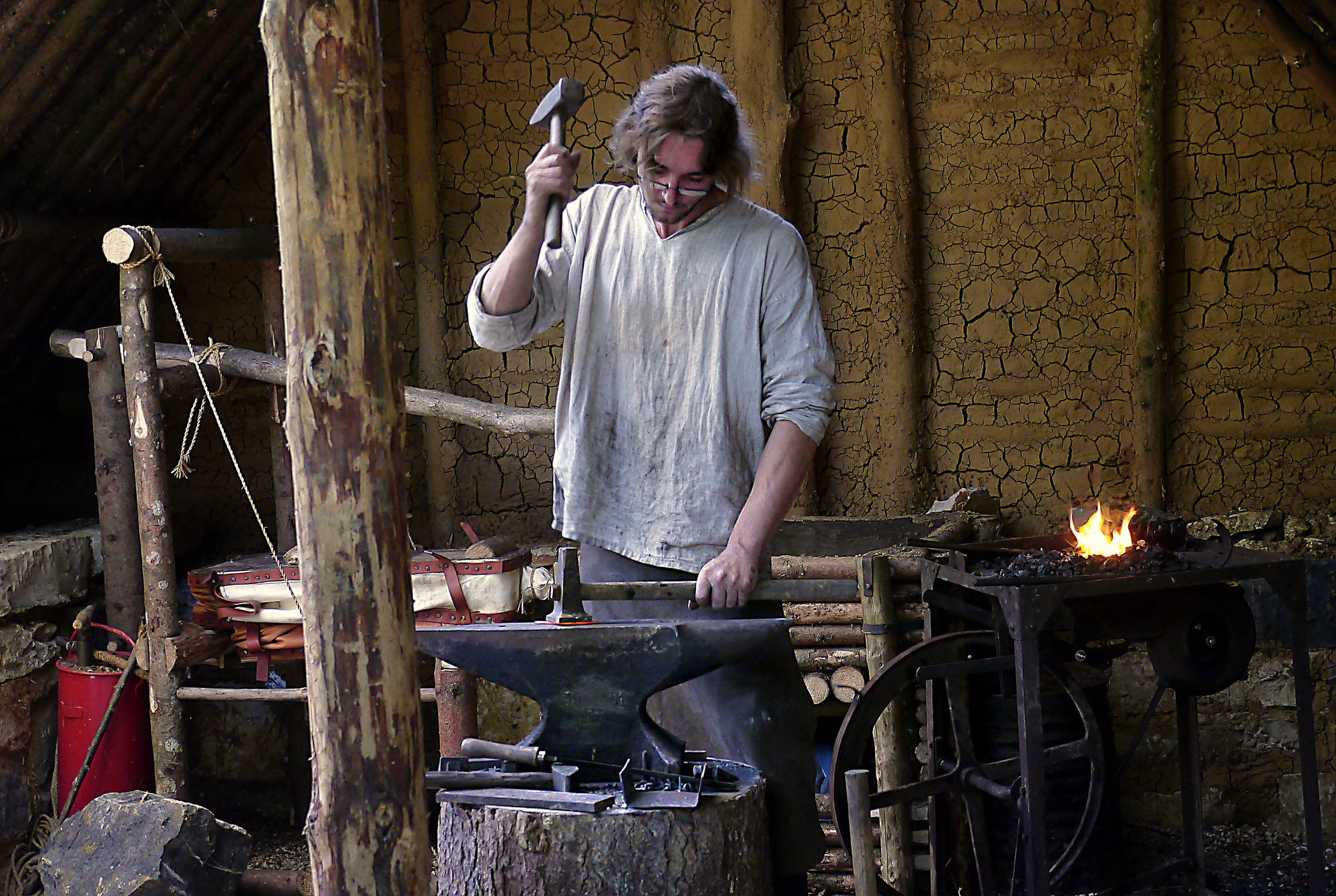A rugged man in his 30s or 40s, with short brown hair and wearing dirty blue pants and a stained white tunic, stands with determination in a dimly lit, medieval-style blacksmith workshop. He is poised mid-strike, holding an object that could be an axe in his left hand while a hammer in his right hand is aimed down at an anvil that rests on a sturdy tree trunk. He wears glasses, emphasizing his focused expression. The surroundings are a mix of coals, a small fire, and a red bucket, with a backdrop of wooden structures resembling a makeshift shed, contributing to the rustic and old-world ambiance. Small, indistinguishable tools scatter the floor near the anvil. The scene is bathed in muted tones of gray, black, brown, and hints of yellow and red, enhancing the historical and handcrafted atmosphere. The photograph, appearing professionally shot, captures the essence of traditional craftsmanship and labor.